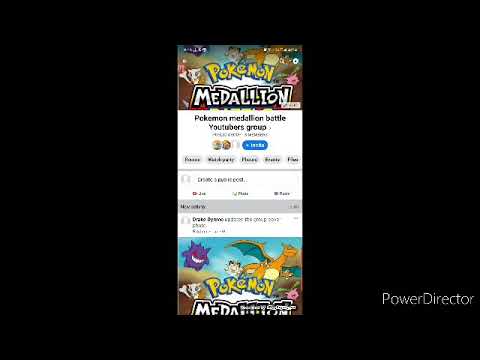The image is a blurred screenshot of a Facebook page against a black background, with "PowerDirector" written in white in the bottom-left corner. Dominating the center of the image is a vertically aligned rectangle displaying a Facebook page for the Pokemon Medallion Battle YouTubers Group. The header features vibrant colors and contains various recognizable Pokémon characters. Although somewhat out of focus, the name "Pokemon Medallion" is clearly written at the top, beneath which is the name of the group, "Pokemon Medallion Battle YouTubers Group." The visible post within the group features an image showing a small purple character with red eyes, a smiling face, a small cat-like Pokémon, and a large dragon-like Pokémon with wide, orange and green wings.